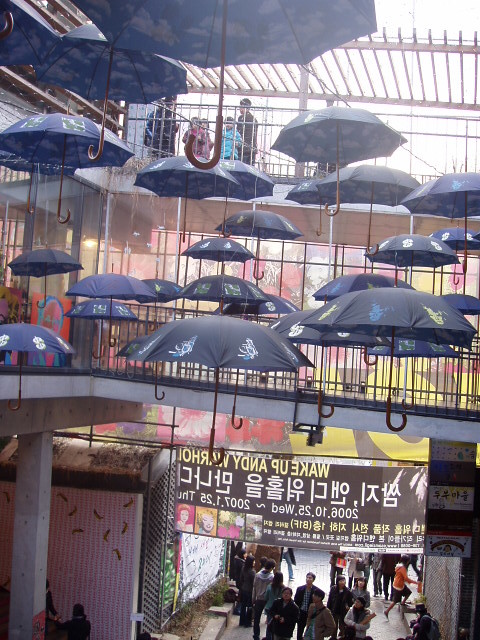The photograph depicts an open-air market or shopping center, likely located in an Asian city such as China, characterized by an overcast sky. The center features three levels with people milling about on each. On the ground level, people walk through a pathway, including a person in a suit and another in an orange shirt. Above this bustling scene, a series of dark navy blue and black umbrellas with unique symbols and Chinese writing are suspended in the air by strings attached to a grated metallic structure. These umbrellas are designed with blue undersides decorated with white clouds, giving the illusion of a sky when viewed from below. On an upper balcony, two adults and three children observe the installation, adding to the communal feel of the scene. A prominent banner hangs above them, featuring both English and Chinese text, announcing an event titled "Wake Up Andy Warhol," suggesting an artistic exhibition or tribute possibly held on January 25th, 2007.